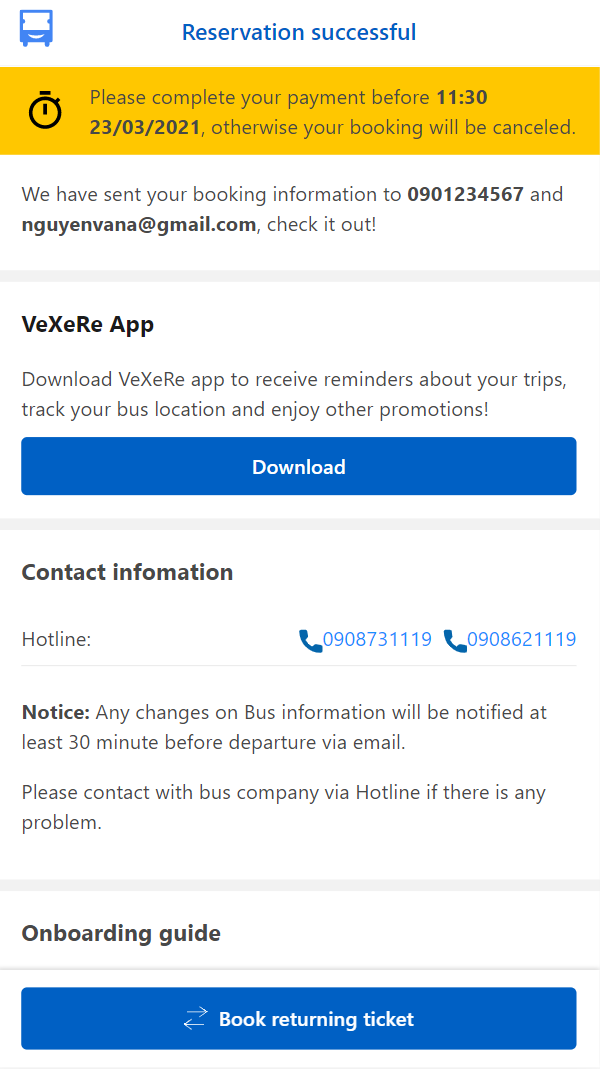**Image Description: Mobile Reservation Confirmation Page**

The image depicts a reservation confirmation page designed in a clean, vertical layout, optimized for mobile viewing. The page lacks typical mobile icons but includes several graphics and information sections.

At the top left corner, there is a playful graphic icon resembling a bus front. This icon features a square, representing the windshield, with two lines beneath it indicating wheels. The bus is illustrated with a whimsical smiley face. The bottom portion of the icon is blue, adorned with a white crescent shape.

Central to the upper banner is the prominent blue text "Reservation Successful."

Below this, a light orange or yellow notification bar features an alarm clock emoji, followed by the critical text: "Please complete your payment before 11:30 23/03/2021. Otherwise your booking will be canceled." This message spans two lines for clarity.

Following the notification bar is a white section containing the text: "We have sent your booking information to 0901234567 and nwinvana@gmail.com. Check it out."

A thick gray dividing line separates this from the subsequent section, which contains a promotion for the "VE XE RE app." Bold black text encourages users to download the app to receive reminders about trips, track bus locations, and enjoy other promotions.

Directly below this text is a full-width blue action button with the white text "Download."

Another gray dividing line segments this section from the next, which provides contact information. The text "Hotline" is followed by two phone numbers on the right side. 

Beneath this is some fine print, advising users that any changes in bus information will be notified at least 30 minutes before departure via email, and instructs them to contact the bus company via the hotline if there are any problems.

Following another gray dividing line, the page features an "Onboarding Guide" section, demarcated by a thin gray line. A blue action button labeled "Book Return Ticket" is located here, adorned with an icon of an arrow (facing right above a leftward arrow) in white, positioned to the left of the text.